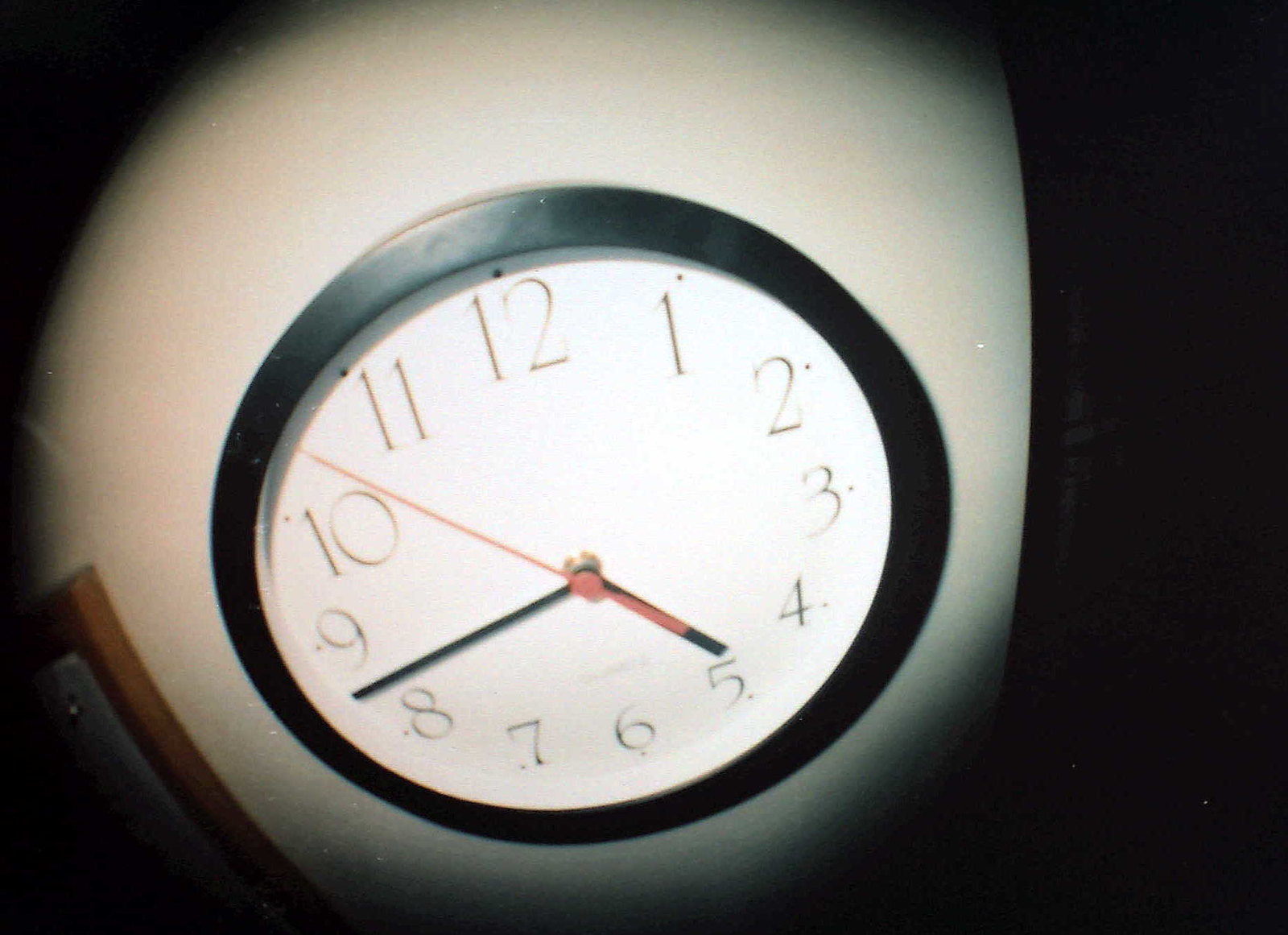The image showcases a simple yet evocative scene centered around a classic, round, analog clock positioned prominently in the foreground. The clock face features black numbers from 1 to 12 arranged in a circle, with the hour and minute hands indicating the time is approximately 4:43, while the second hand hovers between the 10 and 11 marks. Encircling the clock face is a sleek black rim that adds a touch of contrast against the predominantly white wall behind it.

The clock appears to be illuminated by a focused light source, creating a spotlight effect that accentuates its features and casts subtle shadows. This focused lighting underscores the clock as the focal point of the image, causing the surrounding elements to fade into relative obscurity. The white wall on which the clock is mounted recedes into darkness towards its edges, suggesting the scene is set in the corner of a dimly lit room.

In the bottom left corner of the image, there is a small plaque affixed to the wall, which is white with a visible screw securing it to a brown frame. However, this detail is understated, as the primary emphasis remains on the glowing clock face, which holds the viewer's attention firmly within the spotlight.